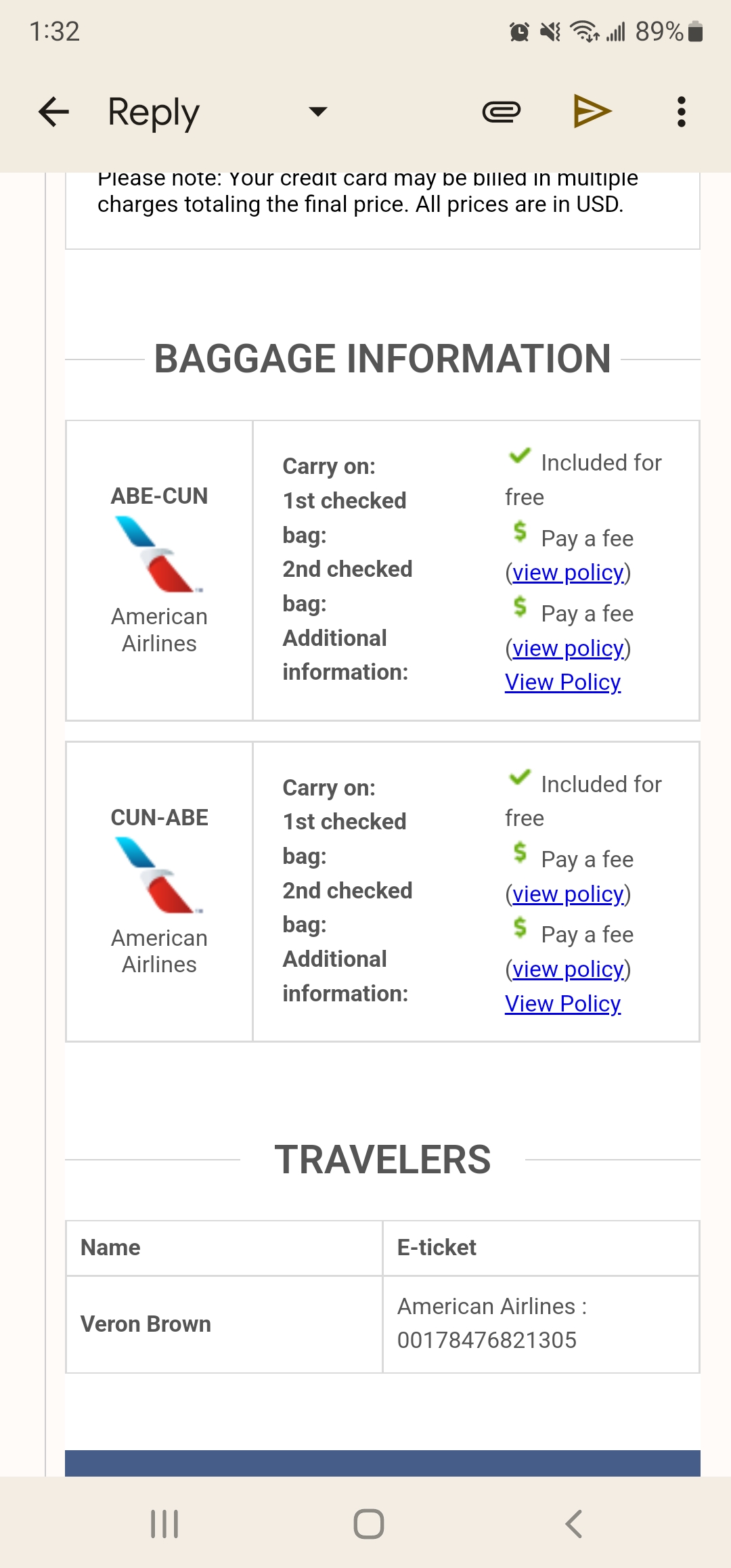The image displays an American Airlines web application on a mobile phone. At the top of the screen, there is a khaki-colored header bar. On the left side of the header, the current time is displayed, while on the right side, there is an 89% battery life indicator, along with Wi-Fi and cellular signal strength icons.

Below the header bar, there is a navigation and function bar. It starts with a "Reply" button indicated by a capital 'R' and a left-pointing arrow. Next to this, there is a document share icon, represented by a paperclip, followed by a "Forward" or "Share" icon, which is depicted as a right-pointing triangle. The last icon in this bar is a "More" option, represented by three vertical dots.

The main content area starts with a notice in black text: "Please note calling your credit card may be billed in multiple charges totaling the final balance. All prices are in USD." Below this notice, there is a section titled "Baggage Information" in capital letters.

The baggage information is presented in two rectangular boxes:

1. The first box is labeled "ABE to CUN," featuring airport codes. It specifies the number of checked bags allowed and what is included. The box also displays the American Airlines logo followed by the text "American Airlines."
  
2. The second box is labeled "CUN to ABE," similarly detailing the return flight information. It shows the American Airlines logo with the "American Airlines" text below it. To the right of this box, there is a square section showing the number of checked bags allowed and what is included for free.

Further below, there is a section for travelers, displaying the traveler's name, "Brown," and the associated e-ticket information for American Airlines.